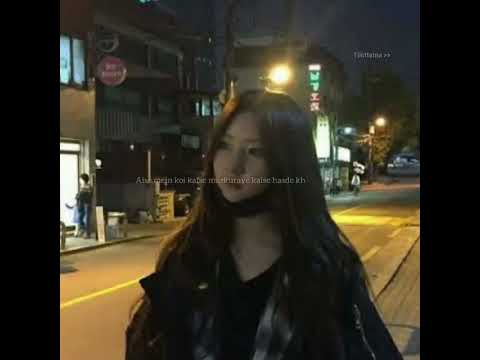In this nighttime urban scene, a woman of likely East Asian descent, possibly Korean, becomes the focal point with her long, dark hair cascading over her shoulders, partially obscuring her clothes. Her expression is one of perplexity and concern as she gazes into the distance towards the left side of the frame. Adorning a black face mask on her chin, she wears a combination that includes a black v-neck shirt, a flannel shirt, and possibly a black leather jacket.

The backdrop paints a vivid picture of city nightlife. Streetlights cast a yellow glow, illuminating a street marked by a solid yellow line. Behind her, a road stretches into the background, flanked by buildings with lit windows and signs, suggesting a bustling area. Some buildings appear tannish, and amidst them, there are also brown benches and alleyways. Text in an unreadable foreign language spans the upper right and across the image, adding to the scene's urban authenticity. The surroundings are dominated by darker hues, such as blacks, grays, and browns, contrasting subtly with occasional splashes of color from signs or lights.

The composition is further framed by black strips on the left and right sides of the image, emphasizing the woman's central position. This detailed capture encapsulates a moment of urban contemplation under the cloak of night, set against a vivid mosaic of city life.